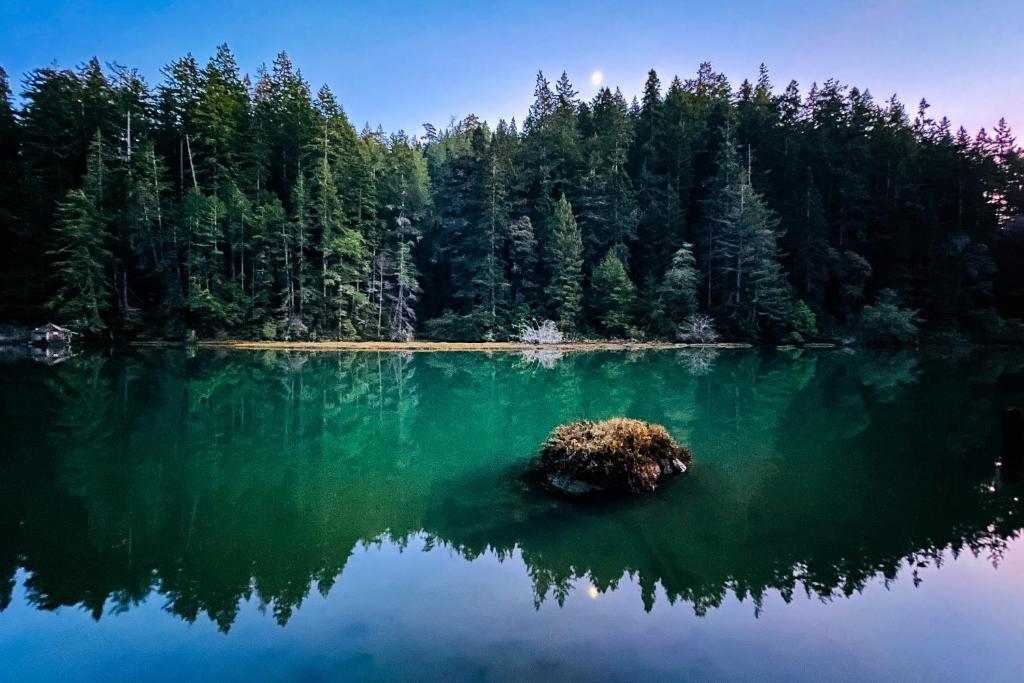The image depicts a serene, still lake with no visible movement on its surface, creating a mirror-like reflection of the towering evergreen trees in the background. The lake's water exhibits a greenish-blue hue, transitioning to a more vivid blue where the reflections of the trees are absent. Centrally placed in the lake is a floating object resembling either a beaver's den or a clump of hay or grass, though its exact nature is unclear. The scene is set against a backdrop of the sky, which shows a deep blue color interspersed with hints of purple, suggesting it might be close to nighttime. The reflections of the trees, sky, and possibly the moon or sun add to the tranquil and picturesque beauty of the scene. Some of the trees in the background appear starkly gray, indicating they might be dead or dying, adding a subtle but striking contrast to the lush greenery surrounding the lake.